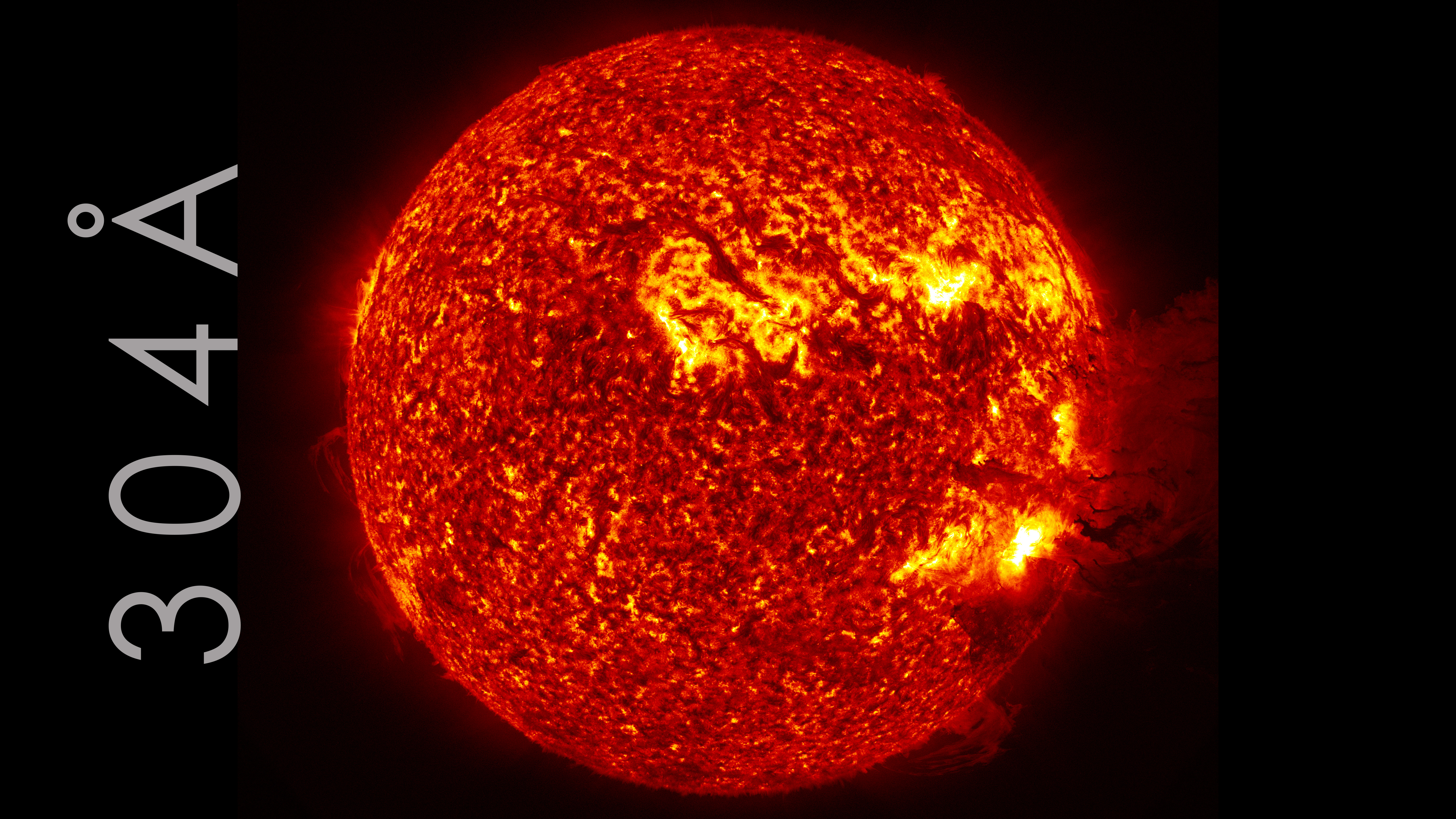This rectangular image, likely taken via satellite or spacecraft, captures a detailed close-up of the Sun in a specific wavelength. The background is entirely black, providing a stark contrast to the vibrant Sun, which is glowing predominantly in dark orange and red hues with brighter yellow spots. Prominently, hot jets of gas, possibly indicative of mass solar eruptions, are seen escaping from the Sun’s surface. Notable among these is a substantial flare shooting off towards the right edge of the frame. Additional smaller streams of gas are visible below and to the left. The image is bordered by two black bars on the left and right. The left bar features the white numbers "304" followed by a stylized "A" with a circle above it, positioned vertically from bottom to top. The Sun appears uniformly round and immensely hot, emphasized by the intense colors and dynamic flares present in the photograph.